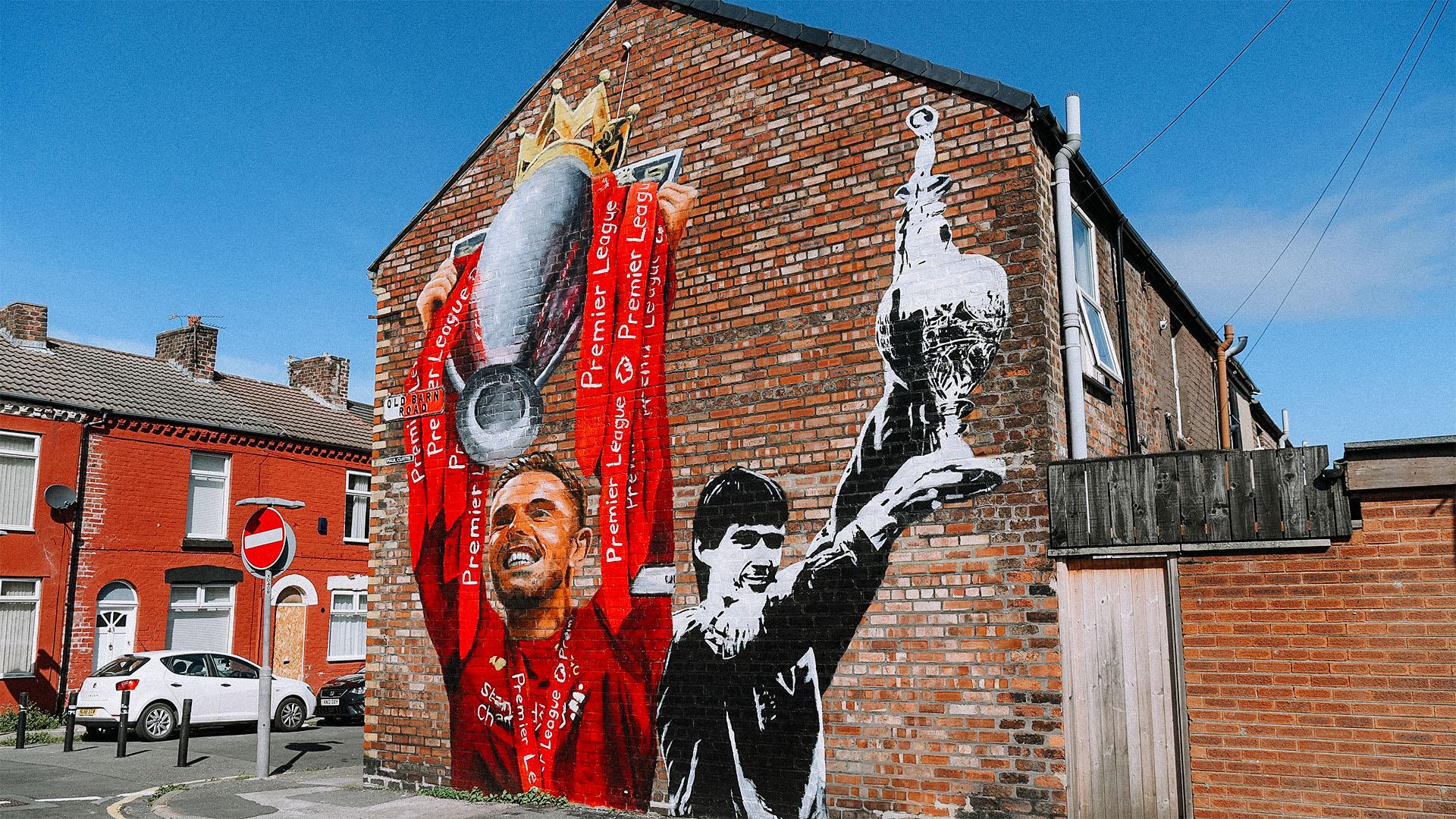This color photograph appears to be taken in the UK and captures an urban setting on a clear, sunny day. Front and center is the side of a multicolored old brick building, prominently featuring a large, vibrant mural that stretches from the sidewalk to near the roof. The mural depicts two soccer players holding trophies aloft. On the left, a player dressed in a red long-sleeved shirt and adorned with Premier League ribbons and a lanyard holds a silver trophy with a gold crown on top. The player on the right is rendered in black and white, wearing a dark uniform, and also holds a silver trophy. This building has a weathered wood balcony attached to it and is windowless on the side displaying the mural.

Adjacent to this building is a row of traditional UK brick row houses in varying shades, complete with chimneys. There is a white car parked on the street in front of these houses. Additionally, a red and white 'No Entry' street sign is situated to the left of the main building. This photograph beautifully combines elements of residential architecture and public art, capturing a snapshot of community pride and culture.